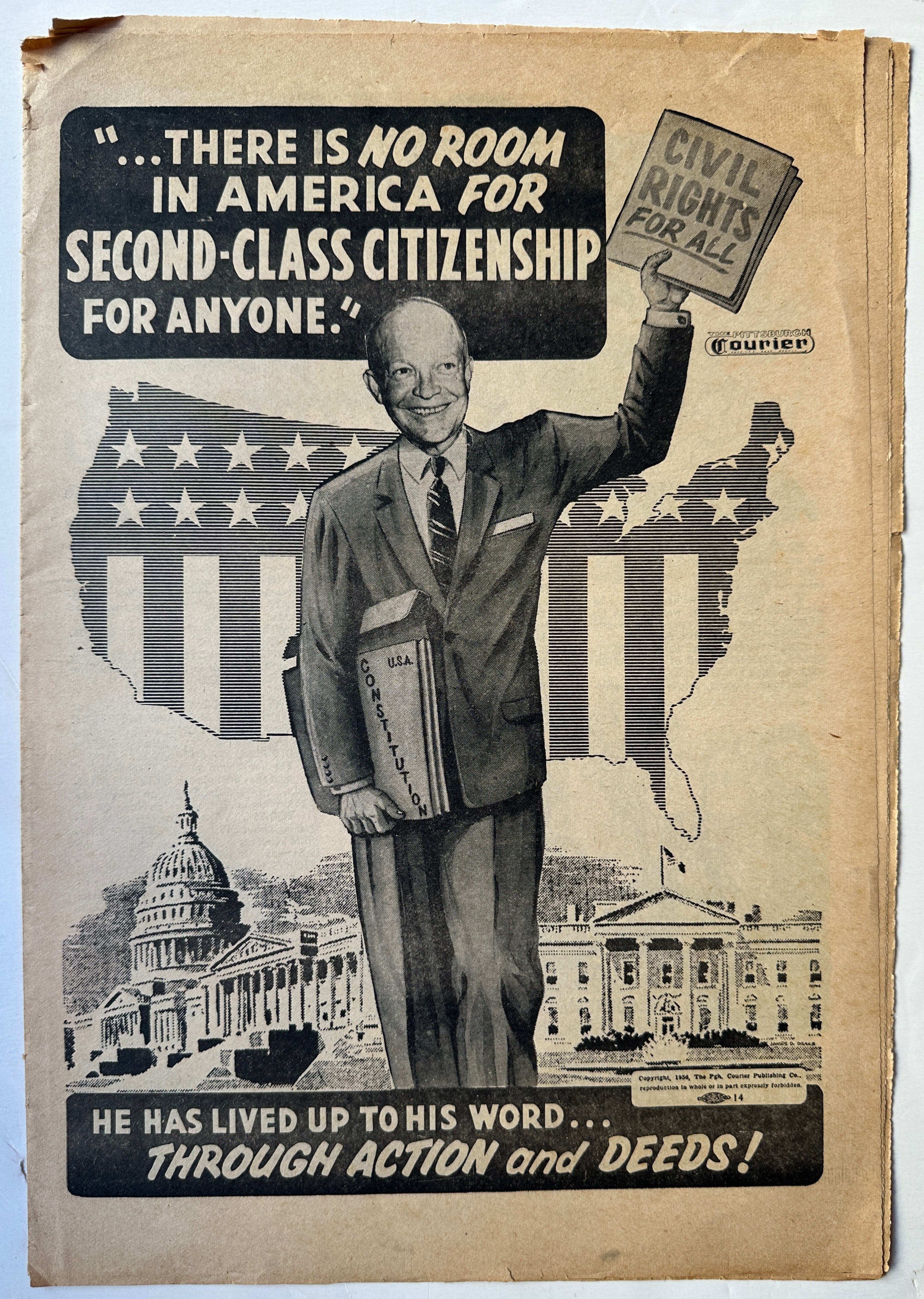This vintage poster on significantly aged and frayed paper features President Dwight D. Eisenhower. The black-and-white image shows Eisenhower, dressed in a suit with a normal tie, holding up a sign that reads "Civil Rights for All." The once white areas of the poster have tarnished to a brown hue. Positioned behind Eisenhower is an emblem of the United States—an outline of the lower 48 states, adorned with stars and stripes as if the flag were superimposed on the map. 

In the upper left corner, on a black background with what used to be white letters, is a bold message: "There is no room in America for second-class citizenship for anyone." This statement serves as a call for equality and good citizenship. In the right-hand corner, there is a small symbol that reads "Courier," presumably the publication responsible for the poster.

Towards the bottom of the poster are black-and-white images of the Capitol Building and the White House, positioned approximately at Eisenhower's knee level. At the bottom, in black with white letters, the text declares, "He has lived up to his word through action and deeds!" This exclamatory statement promotes Eisenhower’s commitment to his policies, suggesting that the poster was likely created to support either his reelection campaign or to affirm his accomplishments during his tenure.